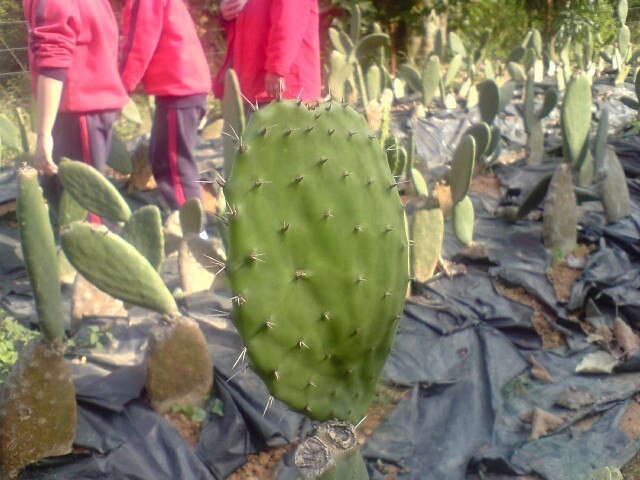In this vibrant outdoor photograph taken on a sunny day, clusters of cacti dominate the scene at what appears to be a cactus farm. The cacti are arranged in rows and surrounded by black plastic tarps utilized for cultivation, emerging from a soil ground. The foreground prominently displays the cactus plants with their spiky leaves, emphasized by the light and shadow cast by the sunlight. To the upper left corner, three individuals dressed in identical outfits—red long-sleeved tops, black pants with a red stripe, and two with additional black arm stripes—are partially visible, facing away or to the side, seemingly walking off toward the edge of the image. The backdrop features trees and bushes against a clear sky, hinting at a serene, rural environment. The colors in the photo are vivid and diverse, including shades of red, black, green, tan, and brown, contributing to the overall natural and lively ambiance of the scene.